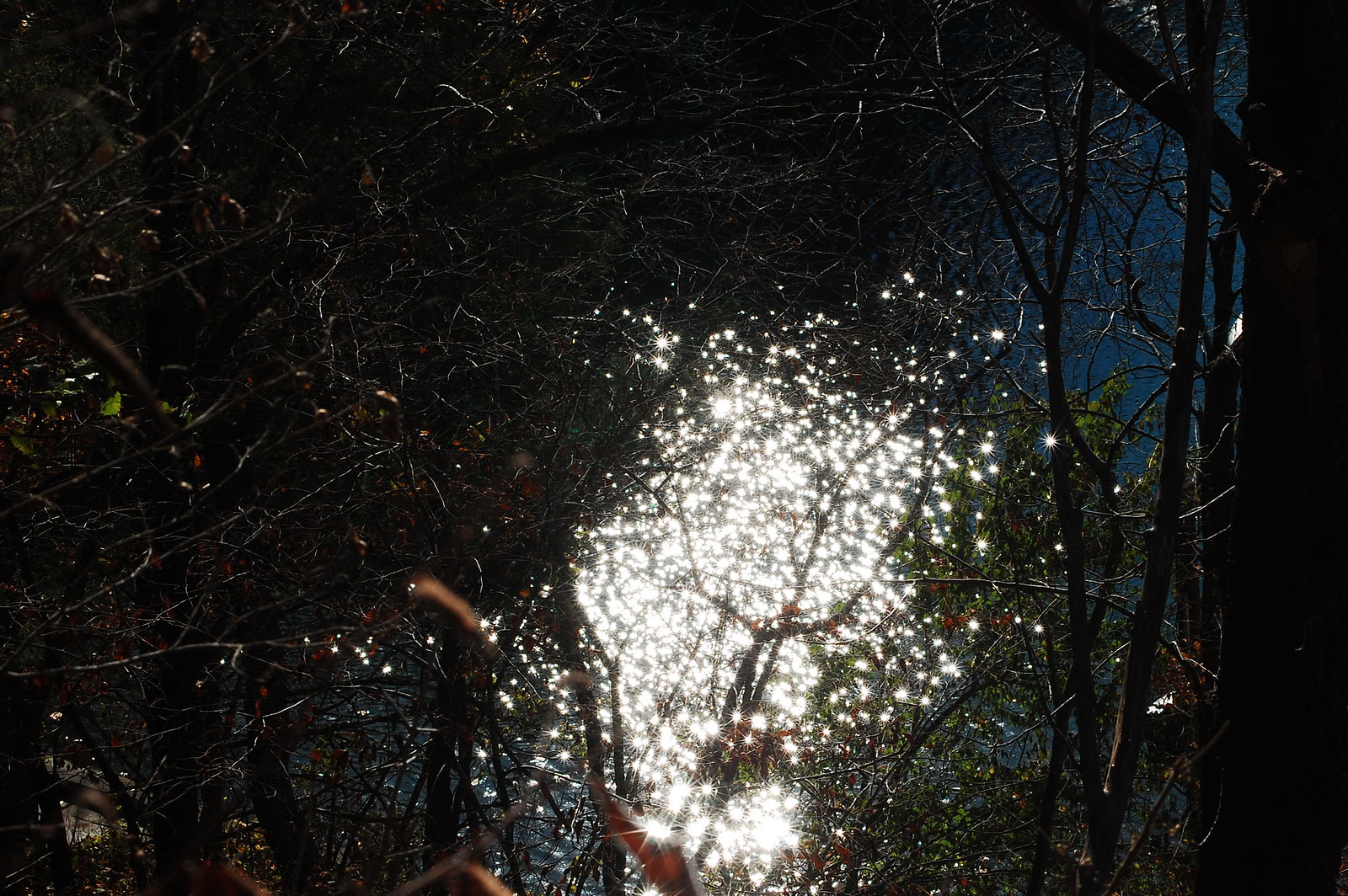The nighttime photograph, rectangular in shape and measuring approximately six inches wide by four inches tall, captures a mesmerizing scene of fireworks. At first glance, the image requires a moment for the eyes to adjust. On the right-hand side, about a tenth of the way in, a dark tree trunk with protruding branches is visible. The left and right sides of the photo are framed by silhouettes of densely packed saplings and tree branches, creating a natural border around the scene. The dark sky, a deep blue hue, contrasts sharply against the bright bursts of light in the center. These light bursts, stretching from the bottom center to the midline, are clusters of white fireworks, sparking and shimmering through the bare branches. The spectacle resembles a mass of tiny, glowing white lights, some clustered together while others stand alone, all creating a captivating display amidst the night foliage. There are no people in the image, just the enchanting interplay between the starlit sky and the firework's brilliance weaving through the trees.